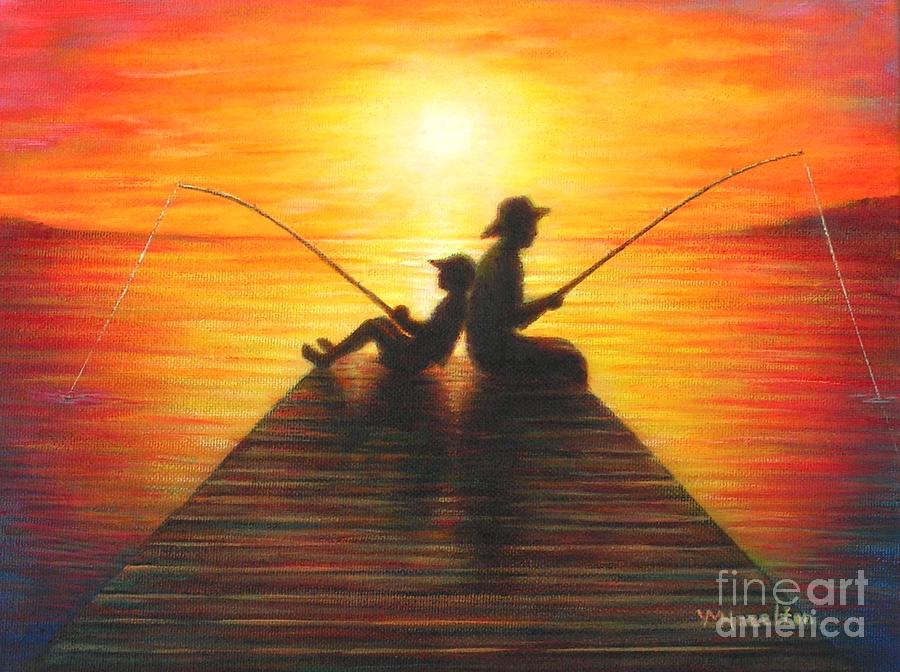The painting depicts two silhouetted figures, one older and one younger, seated back-to-back on the edge of a brown pier during a vibrant sunset. The older figure sits upright, donning a straw hat, with his fishing line cast into the water on the right, while the smaller figure, possibly a child in a baseball cap, leans comfortably against his back, fishing towards the left. The sun hovers just above the waterline, enveloping the scene in brilliant yellows that transition to deep oranges and reds near the edges, casting a warm, nostalgic glow over the water and sky. The pier features subtle hues of light yellow, red, and green. In the lower right-hand corner, the text "Fine Art America" and the artist's signature are visible.